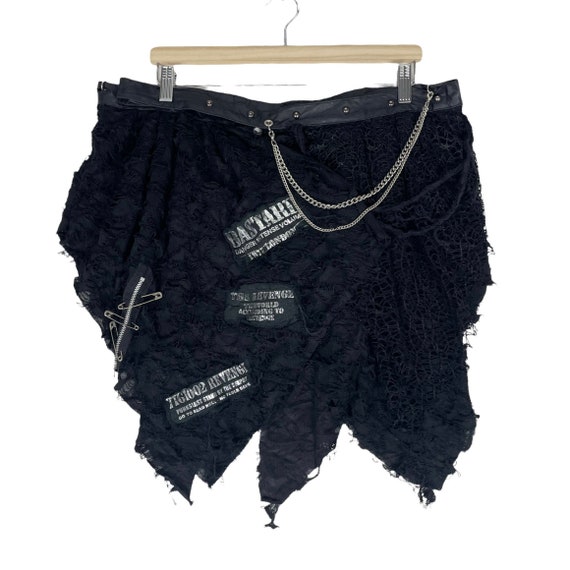The photograph displays a pair of black, heavily distressed shorts hanging on a trouser hanger with two crocodile clips. The shorts feature a ragged appearance with extensive fraying and jagged tears, giving the impression that they have been purposefully weathered. Safety pins are used to hold parts together, particularly noticeable on the left side. The waistband appears to be made of leather and is adorned with metal chains. Additionally, the front of the shorts showcases various patches and badges, including ones that say "revenge" and "bastard." The distressed and punk-inspired fashion is emphasized by the torn edges and the overall ragged look, creating a unique and intentionally worn aesthetic.